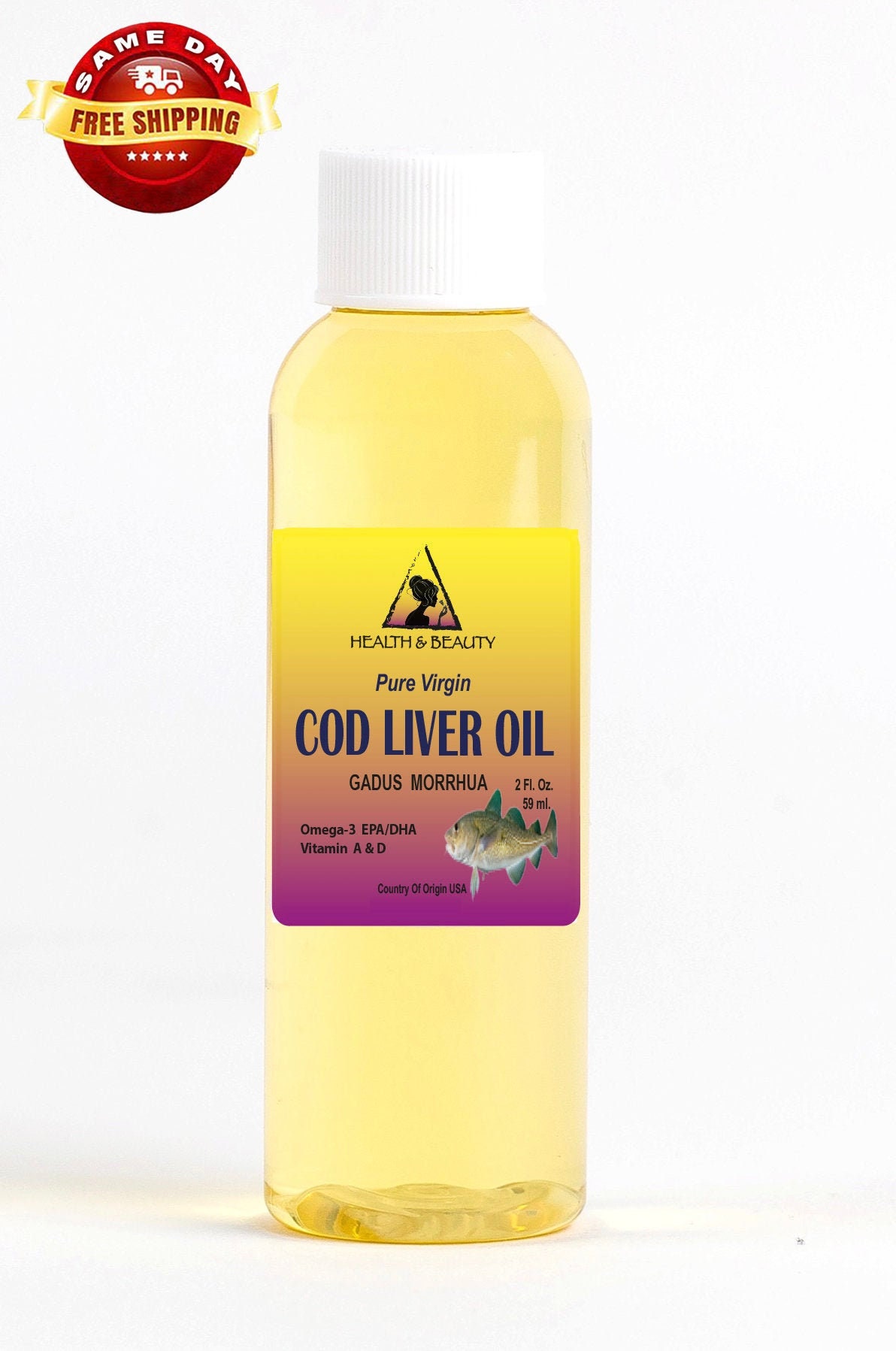This image resembles an advertisement featuring a small, clear plastic bottle filled with yellowish liquid, identified as cod liver oil. The bottle, which has a white screw top, prominently displays a rectangular label that transitions from yellow at the top to purple at the bottom. Dominating the label in bold, uppercase letters is the text "COD LIVER OIL," accompanied by additional information such as "health and beauty," "pure virgin," "two fluid ounces," "omega-3," and "vitamin A and D," though some text remains too small to read. A small picture of a fish is also present on the label. The top left corner of the image features a red circular logo with a yellow banner indicating, "Same day free shipping." The background of the advertisement is a pale gray, and the image is vertically aligned, set against a plain white backdrop.